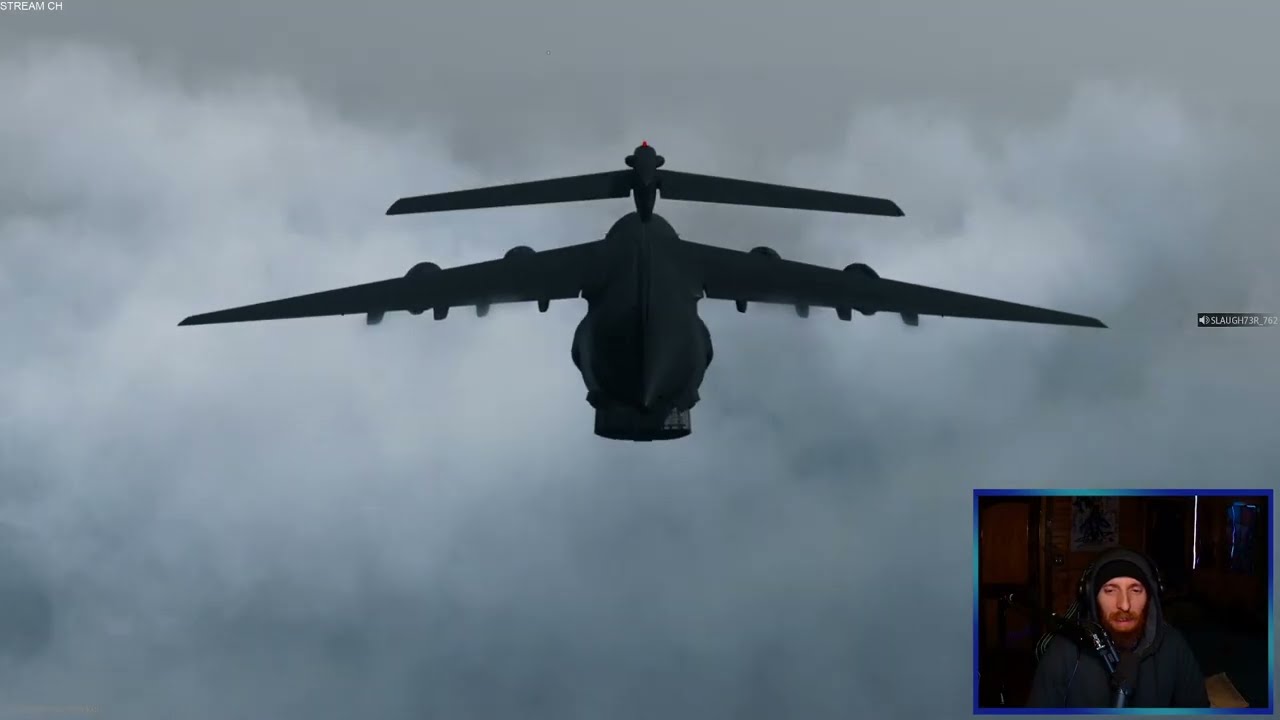The rectangular image is dominated by a large gray airplane flying away through dark, gloomy, gray clouds. The airplane, reminiscent of a military or hover aircraft, has four engines—two on each wing—and features a small tail wing with blades, suggesting some helicopter-like elements. It appears to have a hatch opening at the bottom as it navigates the ominous sky.

In the bottom right-hand corner, there is a small inset image bordered by blue and green alternating colors, depicting a Caucasian man wearing a gray hoodie with the hood over his head. The man has a grayish-red beard and mustache and is seated in a dark room, making the background indistinguishable. The inset indicates that he is either providing commentary or playing a video game, with a microphone symbol pointing to the right accompanied by sound bars and the username "SLAUGH7R_762" in small white letters. This smaller image includes a thumbnail stream channel identifier, "Stream CH", in the upper left corner, further suggesting a live streaming or recorded video setting. The overall composition conveys a blend of aviation and personal engagement through gaming or commentary.